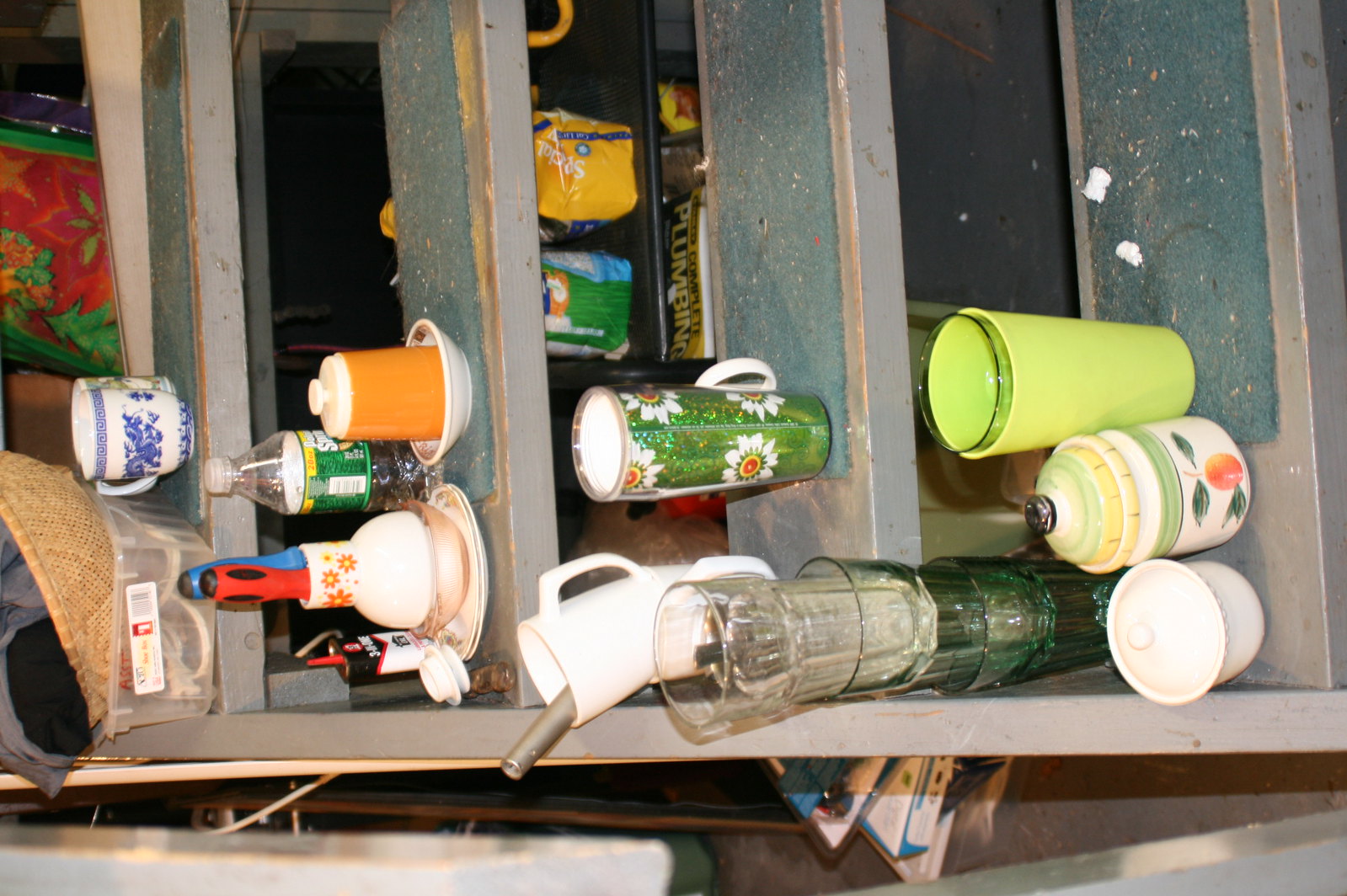Indoor close-up photograph of a set of shelves, rotated 90 degrees counterclockwise. Starting from the bottom, the image shows a horizontal gray wooden piece, now positioned vertically on the left side, which originally forms the side of one of the steps. 

To the left of this gray piece and on the first shelf, there is a green Tupperware container holding a basket. Beside it, toward the right side of the shelf, stands a ceramic coffee cup with blue printing.

Moving rightward to the next shelf, we see a collection of white ceramic saucers and plates. Also on this shelf are an empty bottle that appears to be Sprite, a couple of lint rollers, and a small can of 3-in-1 motor oil.

On the subsequent shelf to the right, a tumbler adorned with a green label and white flowers is positioned. Next to this tumbler, there are two ceramic coffee cups stacked on top of each other, with a cylindrical object protruding and pointing downward.

Finally, on the last shelf to the far right, there is a stack of four or five drinking glasses. Additionally, we spot a white ceramic saucer, a cookie jar, and a green cup.

In the background, visible through the gaps in the shelves, there seems to be a bag of peat moss or cat food. Near the bottom left side of the image, through the wood, one can see some white and blue boxes stacked together. No visible words, text, or print appear in the photograph.